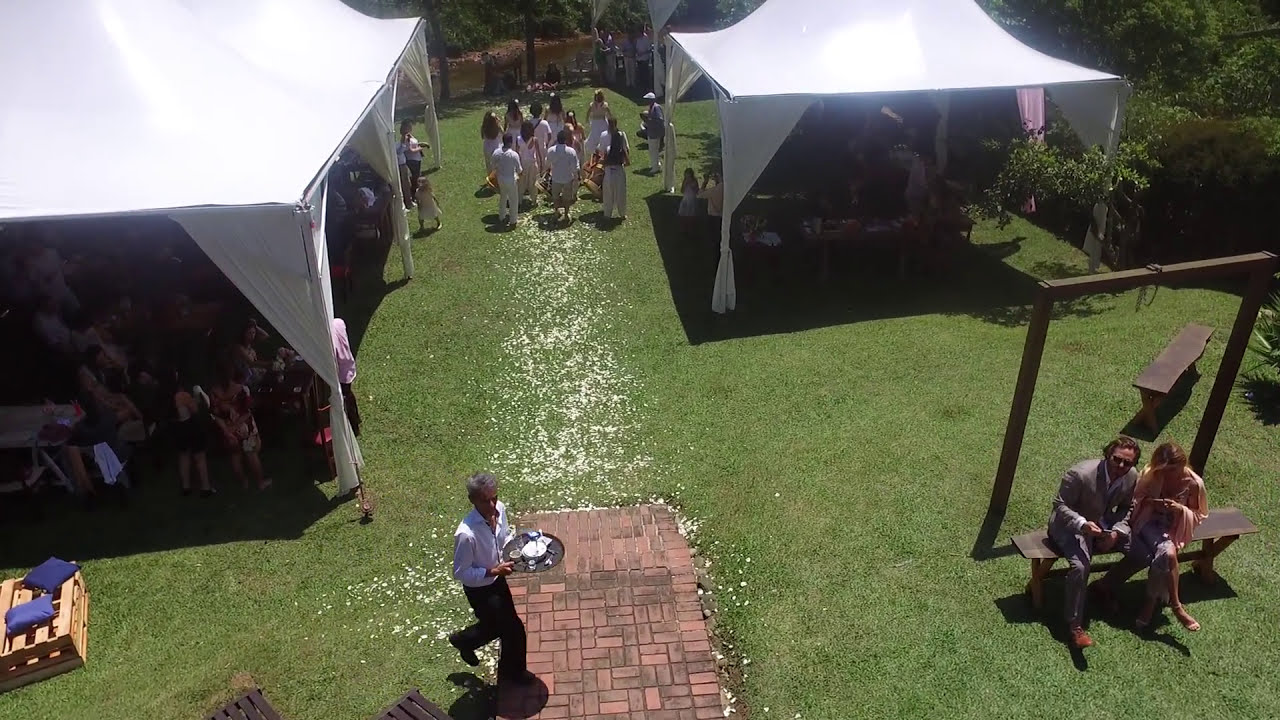This vivid aerial photograph captures a joyous outdoor wedding reception set amidst a serene and lush green lawn. Dominating the scene are two white canopy tents situated on opposite sides of a small, paved walkway, one to the left and one to the right. Beneath these tents, formally dressed guests are seated, their conversations and celebrations adding to the lively atmosphere. In the foreground, a waiter distinguished by his white shirt and black pants carries a silver tray laden with food, navigating the gathering with ease. To the right, a young couple shares a peaceful moment on a wooden bench. At the end of the walkway, a larger congregation, possibly participating in a ceremonial activity, adds to the scene's dynamic energy. The entire area is embraced by verdant bushes and towering trees, creating an idyllic setting perfect for such a beautiful, sunlit event.